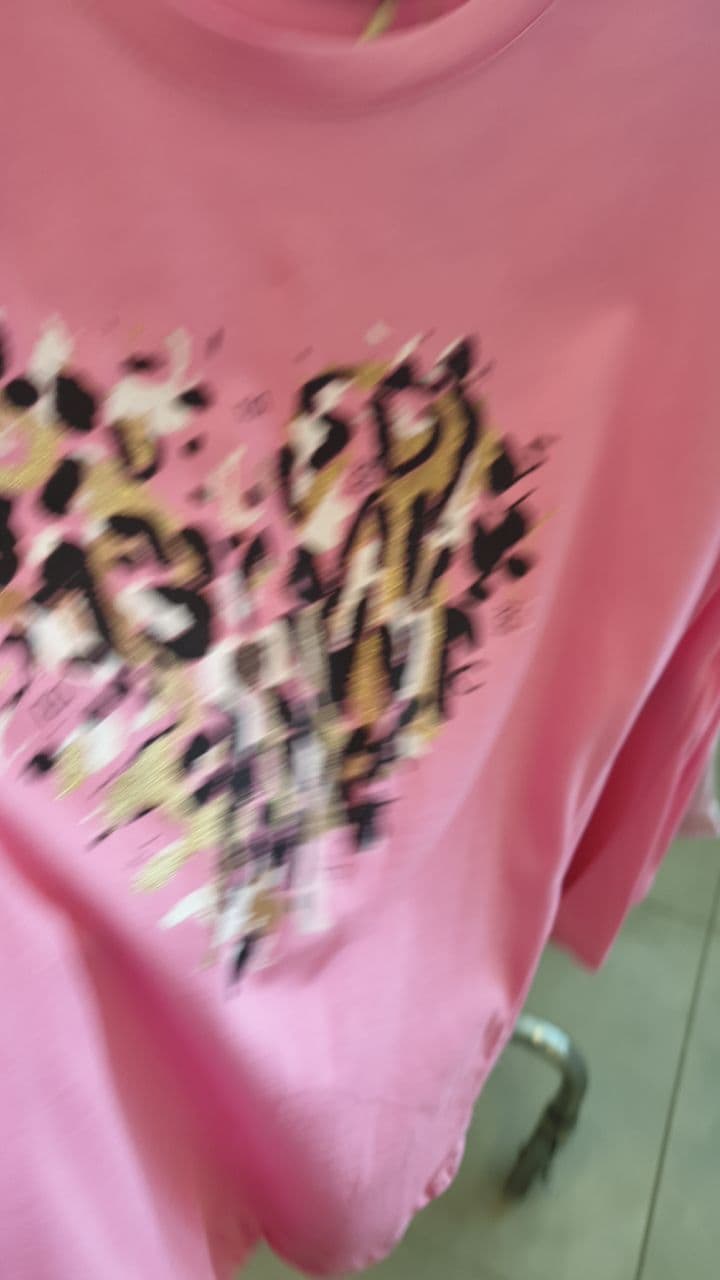The image is a detailed, well-lit, but slightly out-of-focus indoor photograph that looks down on a pink women's long-sleeve shirt draped over a shiny chrome rack, likely in a clothing store. The high vantage point captures a pattern forming a distinctive heart shape in the center of the shirt, featuring streaks and splatters of black, white, gold, and brown paint, resembling a colorful paint-splatter or abstract leopard print. The shirt appears to be brand new, with no tags visible. Some portion of the left sleeve is hanging just below center on the left edge of the frame. In the bottom corner, part of the chrome base of the rack and its gray wheel, complete with a locking mechanism, are visible, resting on a tan tile floor, typical of a store environment.